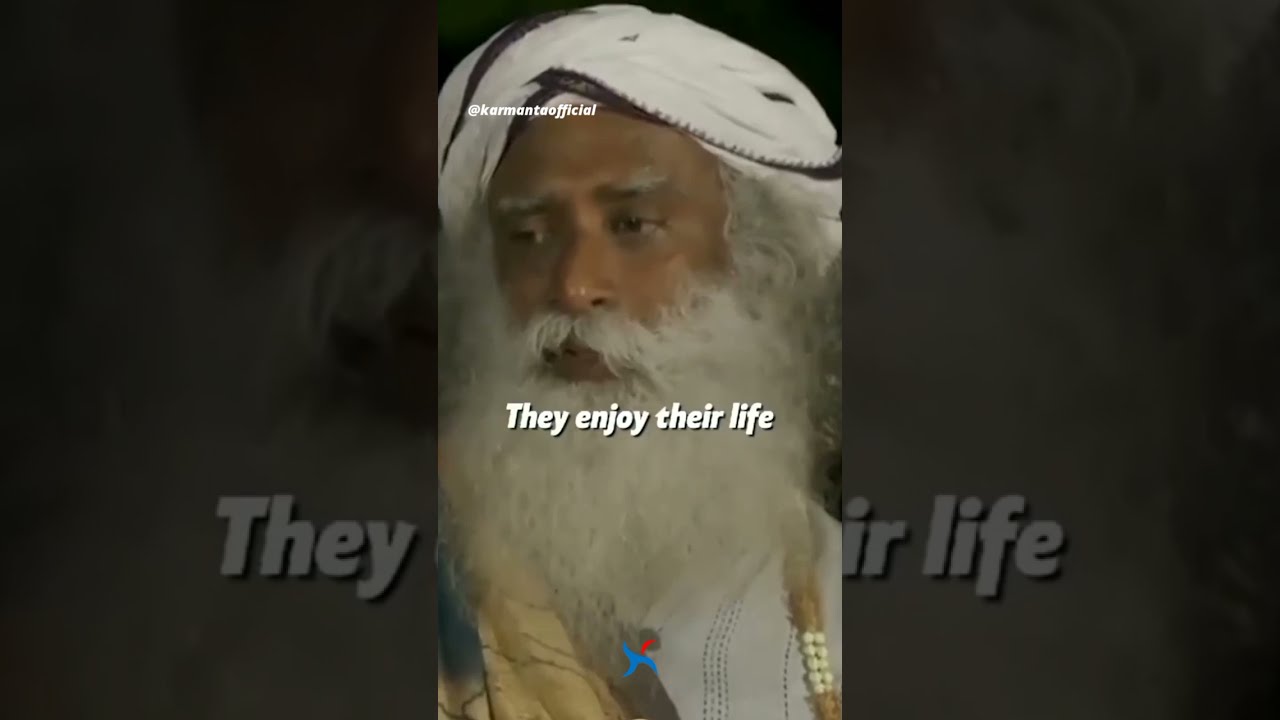The image depicts an older man, likely of Middle Eastern or Arab descent, characterized by his long, white beard and mustache that covers most of his face, reminiscent of Santa Claus. He wears a distinctive white hat, which may be of religious significance, and a tan-colored robe layered over a white shirt. His hair, adorned with white beads, partially falls to the side. The central focus of the image is the text that reads "They enjoy their life" in bold white letters. Additionally, there is a social media handle, @KarmanTaoOfficial, featured prominently in the top left corner. The image also includes a blue squiggly line logo at the bottom center. The background is minimal, ensuring emphasis remains on the man and the text.